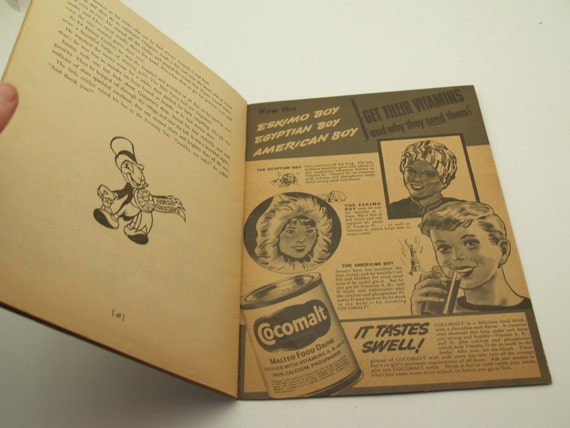The image captures an old, black-and-white booklet with yellowed, faded light brown pages, resting on a white tabletop indoors. A person's hand, positioned on the left, holds the booklet open, revealing two pages. The left page features text in the upper section and an illustration of Jiminy Cricket from Disney's "Pinocchio." The right page displays an advertisement for a malted food drink called Cocomalt. The ad prominently shows a tin can labeled "Cocomalt," accompanied by illustrations of three boys: an Eskimo boy with a furry hood resembling someone of Asian descent, an Egyptian boy with dark brownish skin, and an American boy with classic white features and blonde hair. They are all depicted drinking Cocomalt. The text describes how these boys get their vitamins and why they need them, highlighting the drink's nutritional benefits.